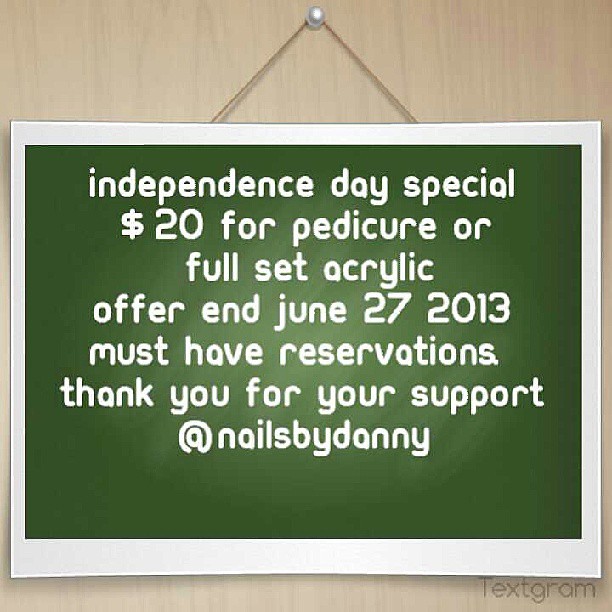The image depicts a computer-generated, cartoony graphic created with a program called Textgram. It features a light wood wall background, on which a green blackboard with a white border is hanging from a shiny white push pin. The text on the green blackboard, all in lowercase and without punctuation except for a period after "reservations," reads: "independence day special. $20 for pedicure or full set acrylic. offer end june 27, 2013. must have reservations. thank you for your support. at nails by danny." In the bottom right corner of the image, there is a small, gray watermark that says "Textgram." The entire graphic appears to be 6 inches wide by 7 inches tall and conveys a handmade feel, though it is digitally created. There are no other objects, contact information, or additional details provided in the advertisement.